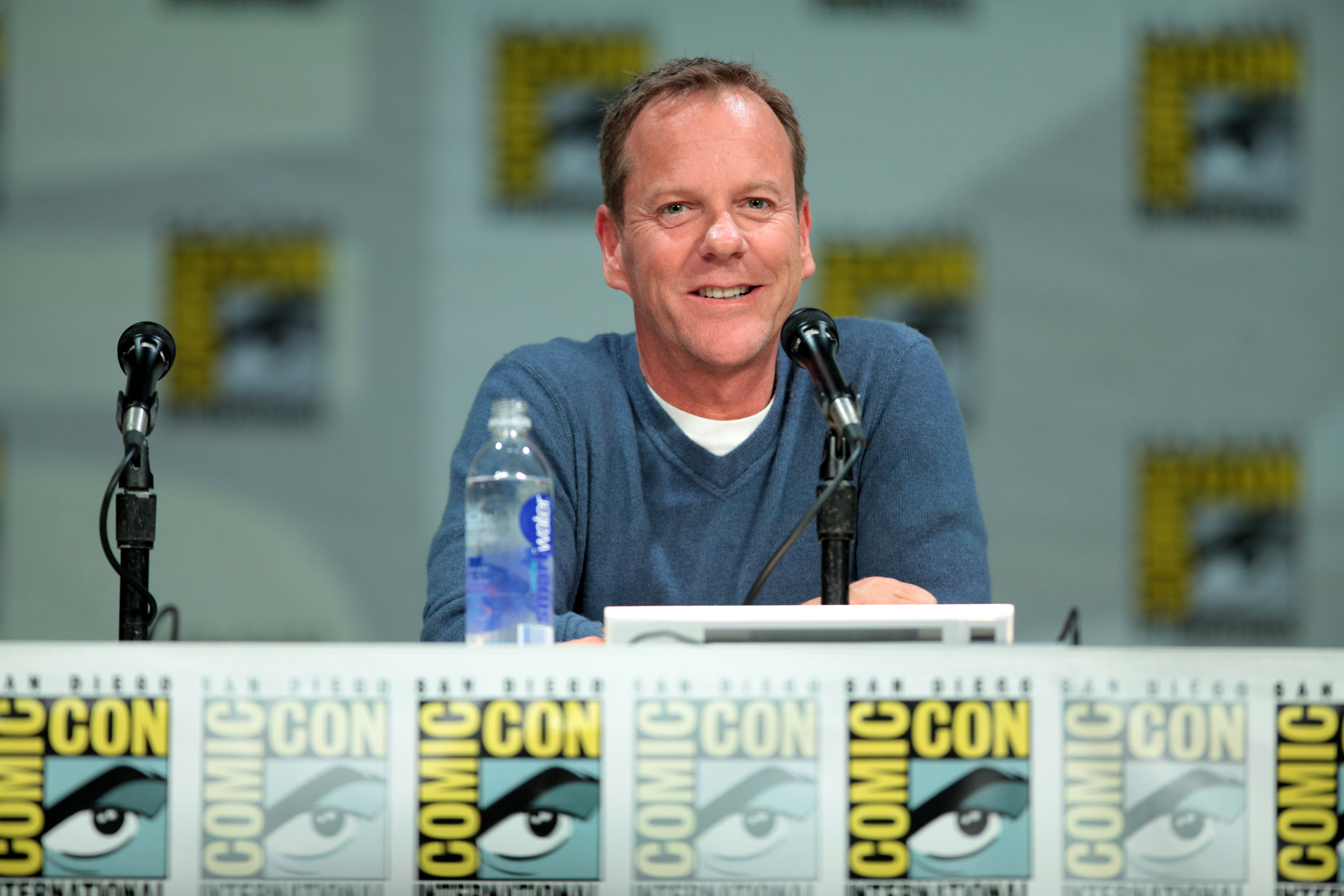This detailed photograph captures actor Kiefer Sutherland at San Diego Comic-Con, sitting at a long table that extends out of the frame, thus isolating him in focus. He wears a blue V-neck sweater over a white shirt and leans slightly forward with his hands crossed together on the table. A black wired microphone is positioned in front of him, alongside a three-quarters full Smartwater bottle. Another unused microphone is placed near him on the table. 

Sutherland appears to have just answered a question, as he looks ahead with a reflective expression, his slightly crooked nose and subtle wrinkles showing signs of middle age. His short brown hair has a slight faded shine. Behind him, the iconic Comic-Con logo forms a blurred backdrop, while directly in front of him, a banner displaying the San Diego Comic-Con International logo with the distinctive eye motif is visible. His demeanor suggests engagement, with eyes that hint at reacting to a thoughtful question from the audience.